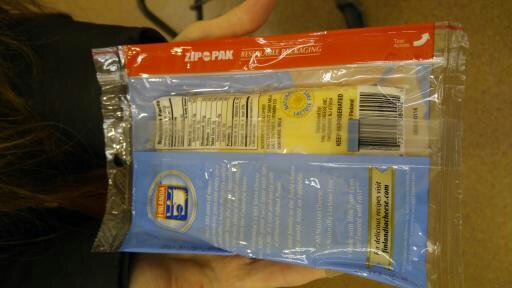The close-up image features a person holding a packaged food product wrapped in cellophane. The rectangular package, labeled "Zip Pack" in a red stripe at its upper part, is designed with a zip closure. The package is held in both hands and appears horizontally oriented, though the text is vertically aligned. Below the Zip Pack label, the package displays nutritional information on a white background, followed by a yellow label, and a UPC code directly underneath it.

Further down, the packaging includes marketing information about the product, presented on a blue background with white text. A logo is positioned at the top of this section, while a yellow ribbon graphic suggests that additional information can be found on the product’s website.

The person holding the package is standing on a beige floor which seems to be either tiled or made of linoleum. The person’s attire consists of black clothing, providing a stark contrast to the floor and the package they are holding.